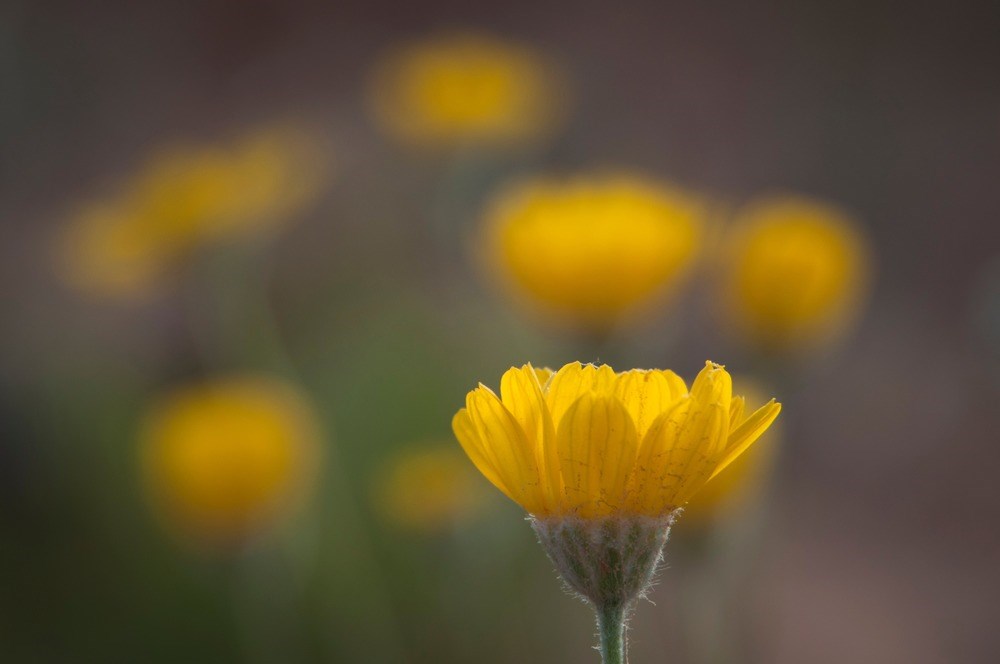This horizontal photograph captures an up-close, detailed view of a single yellow flower positioned in the lower right quadrant of the image. The main subject is a side view of the flower, showcasing around ten vibrant yellow petals. The base of the flower features a green, V-shaped structure with a visible stem that is partially cropped at the bottom. The background is intentionally blurred, creating a stark contrast with the sharp focus on the foreground flower. In this blurred backdrop, various shapes and colors can be discerned, including the outlines of at least six other yellow blossoms and some green foliage, set against a dark, grayish-brown haze. This photographic composition suggests a natural, outdoor setting, with the use of depth of field emphasizing the single flower amidst a softly muted, indistinct garden landscape.